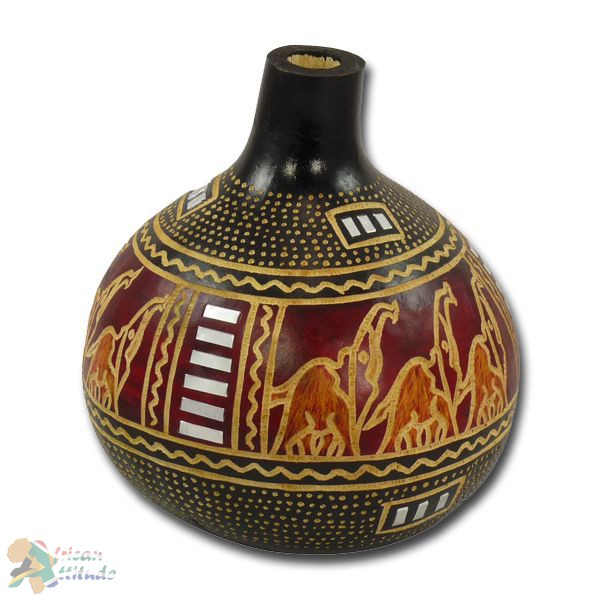The image displays an intricately hand-painted artifact, likely of African origin, resembling a round jug or vase with a small aperture at the top, reminiscent of an upside-down light bulb. The object, possibly made of wood or gourd-like pottery, features a predominantly black base adorned with gold stipple work and delicate lines. Central to its design is a deep red band encircling the middle, depicting what appear to be animal outlines, potentially elephants, rendered with fine detail. The motif evokes the style of Greek statuary, with animals positioned counterclockwise around the pot's circumference. The top section mirrors the bottom with its black and gold patterning, except for the entirely black neck of the vessel. Positioned at the bottom left of the image is a colorful logo bearing the phrase "African Attitude," incorporating a large, stylized "A" overlaid with the African continent. Set against a pure white background, this photograph seems intended for retail display.